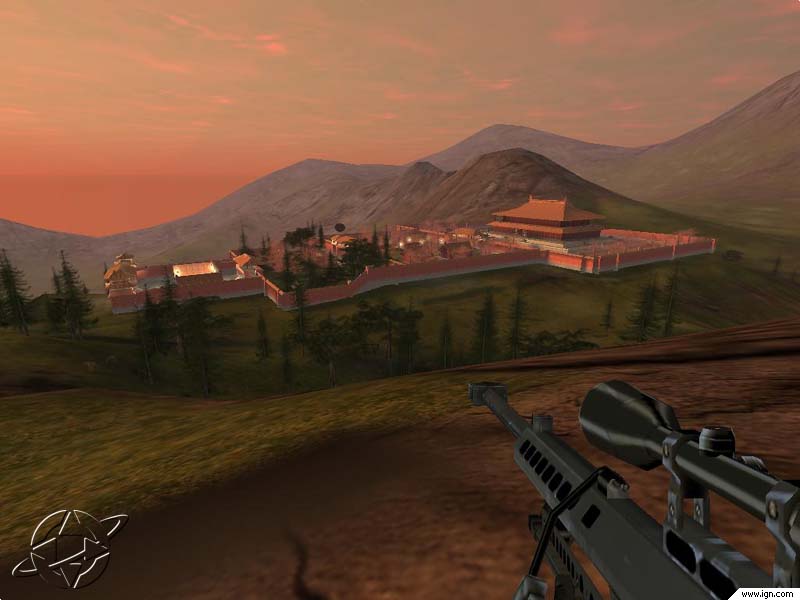This image, likely a screenshot from a first-person shooter video game, showcases a tranquil yet suspenseful scene at dusk. The view, slightly wider than it is tall, features a black, scoped rifle in the lower right-hand corner, peeking into the frame as if being readied by the unseen character. The foreground consists of reddish-brown dirt transitioning into green, grassy terrain on a slight incline. The character appears to be positioned on a hill overlooking a scenic valley filled with a mixture of greenery and sparse trees.

Dominating the midground is a fortress-like compound with distinctive Asian architectural elements, including sloped, layered roofs on its buildings. This compound is surrounded by a prominent, pinkish-red brick wall. The largest building, central in the image, catches the eye, accompanied by other smaller structures within the walls. The backdrop reveals a series of gentle, sloping mountains, enhancing the sense of depth and scale. The sky, painted in shades of orange and pinkish-blue, suggests a setting sun, casting its warm glow over the serene and expansive landscape. In the bottom right corner, subtle text reading "www.ign.com" confirms the image's video game affiliation.